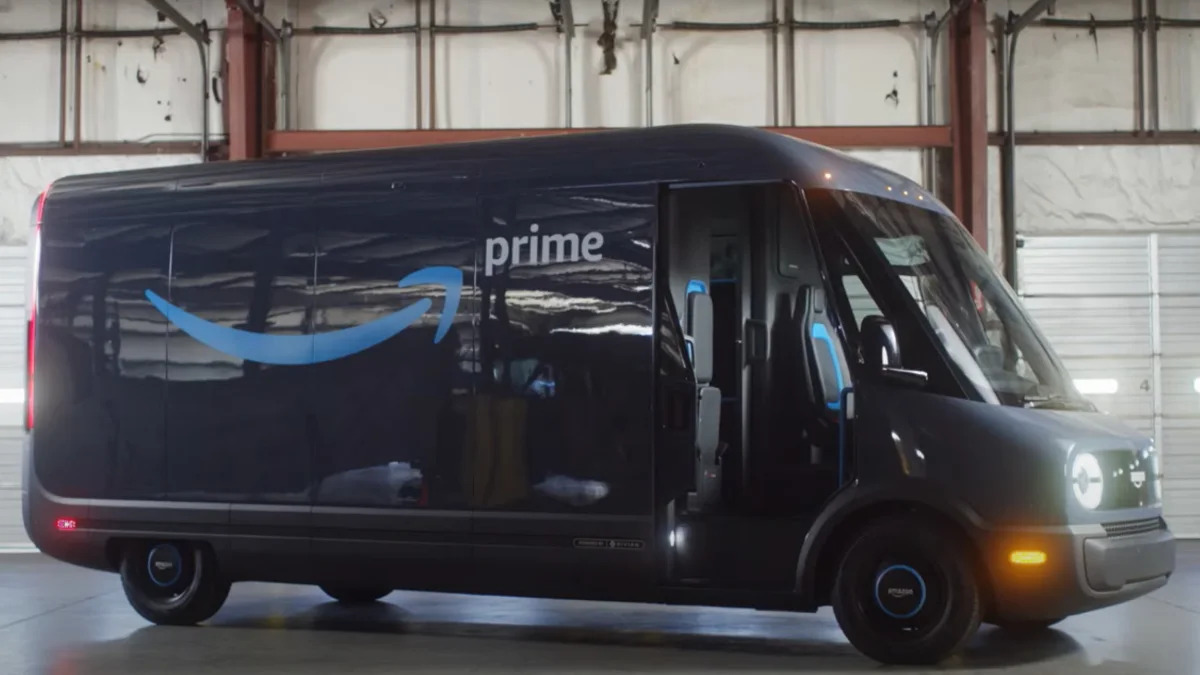In the image, an Amazon Prime van is parked inside a spacious, well-lit parking garage. The van is notably long, with its cab pointed towards the right side of the image. The polished exterior of the van gleams under the lights, prominently displaying the Amazon Prime logo. The headlights are illuminated, including an orange, rounded rectangular light positioned near the bumper.

The van's wheels are modern and feature an Amazon-themed icon at the center, where the hubcaps would typically be. The side door is open, hinting that it might be a sliding door or simply designed to stay open. The visible seat resembles a high-end gamer's chair, featuring modern ergonomic design with light blue accents supporting the backrest.

Through the open door, part of the van's cargo area is visible, revealing two blue-outlined, rectangular panels that appear removable. The garage itself has white walls and steel beams with a reddish hue forming the structural framework. These beams create an H-shaped structure visible behind the van. To the right, behind the van’s engine section, a garage door is seen, characterized by five horizontal rows and two vertical columns of panels, with two thin openings in the middle row.

The floor of the warehouse is constructed from gray concrete, with the van casting a small shadow on it. Red taillights at the back of the van add a splash of color amidst the otherwise neutral tones of the environment. Overall, the image captures the sleek and functional design of the Amazon Prime van against the industrial backdrop of the parking garage.